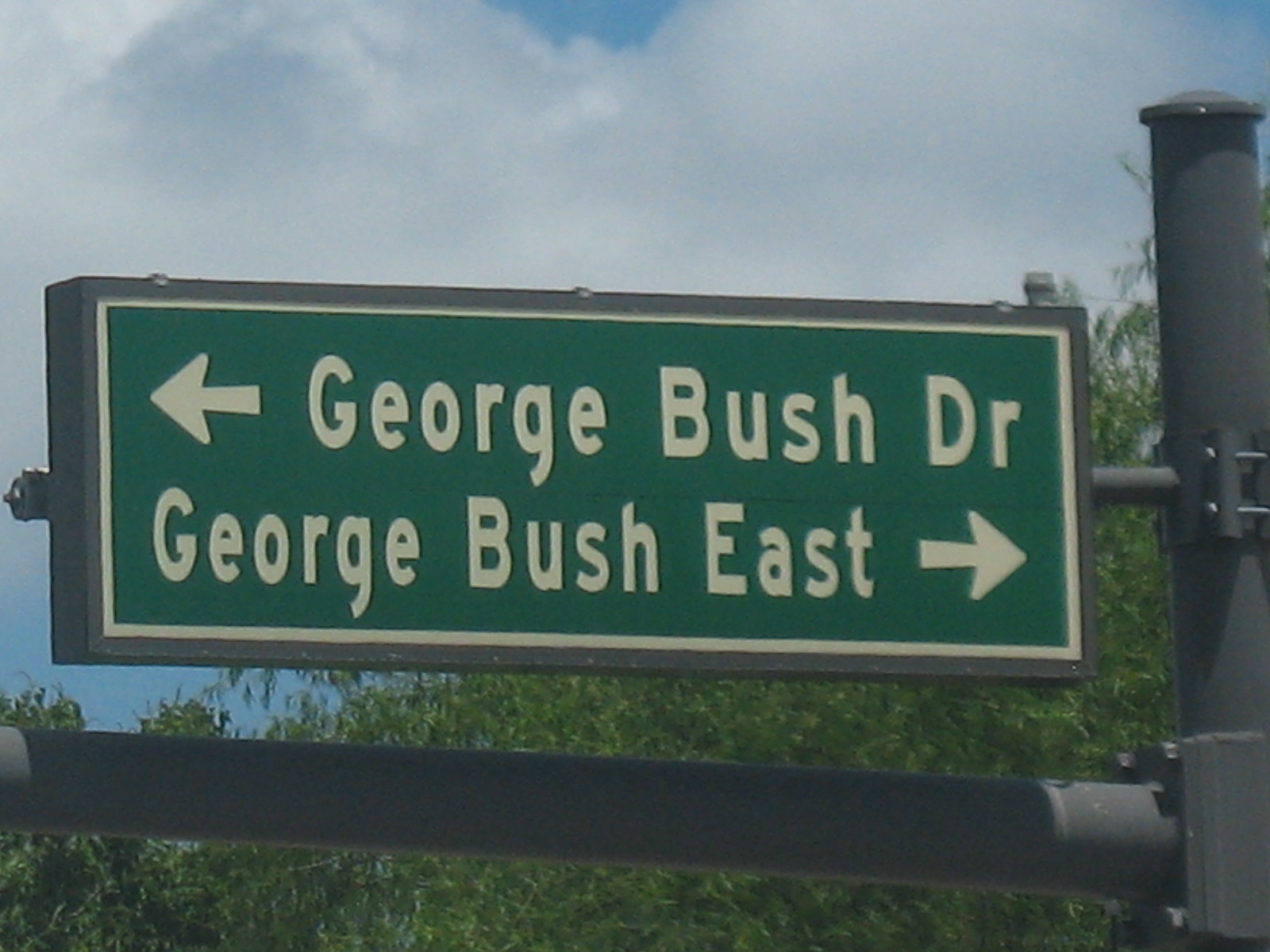The image captures a detailed view of a street sign mounted on a dark gray, almost charcoal, metal pole. This pole features a vertical section visible on the right-hand side and is accompanied by horizontal extensions; one near the bottom of the image and the other in the center. The central horizontal pole is slimmer and holds the key street sign. The sign itself is square-shaped with a dark charcoal gray exterior border, followed by a cream-colored inner border encasing a forest green background. The street sign displays two directional arrows: one pointing left with the inscription "George Bush Drive" and the other pointing right labeled "George Bush East," both written in a cream color. 

The scene is set against a backdrop of a blue sky adorned with fluffy white and gray clouds. Below the sky, the tops of lush, green trees add a touch of natural beauty. The image also hints at additional infrastructure below the main street sign, likely another horizontal pole extending from the vertical one, possibly intended for a traffic light, though that light is not visible in the frame.